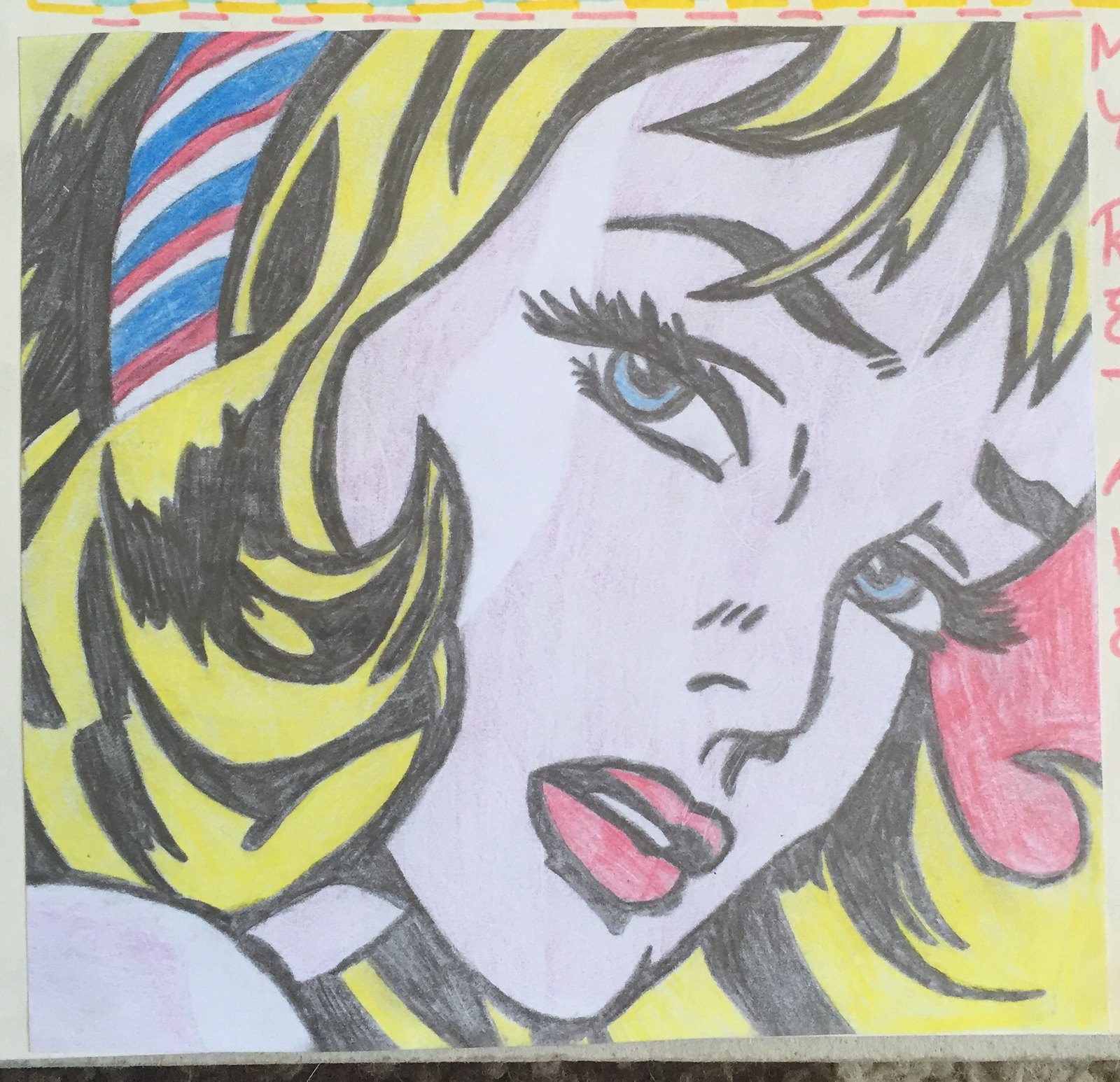The image captures an extreme close-up, detailed colored pencil or crayon drawing of a woman's face. Her head is tilted slightly diagonal, composed with a palette of red, white, blue, yellow, pink, and black hues. She dons a red, white, and blue striped headband woven through her yellow-blonde hair that's outlined in black, with strands falling onto her cheek. Her piercing blue eyes, defined by black pupils and lashes, gaze directly at the viewer, while her lips, shaded pinkish-red and outlined in black, are slightly parted revealing a hint of white. Her nose is subtly outlined with black for definition. At the bottom left, the tip of her right shoulder appears with a light grey hue while a small grey neck transitions to her meticulously shaded face. The background features varying shades of yellow and hints of black that likely represent her hair. The left side reveals a gray, circular form, probably her shoulder. The image shows a pink and yellow dotted line along the top frame and a mysterious red mark on the lower right. The entire artwork is situated on what seems to be a tan felt backdrop, suggesting the piece might either be a poster or wall art.